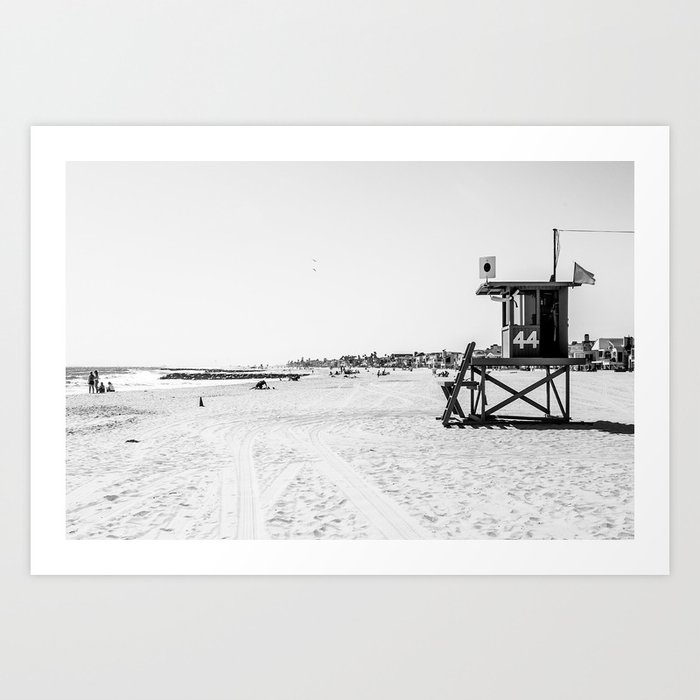The image features a larger square light gray frame with a white-bordered, horizontal rectangular photograph in black and white at its center. The scene captured is a sandy beach with numerous vehicle tracks, and to the left, the shoreline touches the ocean. Prominently positioned on the right side of the image is an elevated lifeguard shack, simply constructed with a framework of boards and marked with the number 44. Several small flags flutter from the shack, and there's a silhouette of a person's head visible within it. Below, a ladder leads up to two separate outdoor sitting areas for lifeguards. In the extreme left background, a row of buildings, presumably beach houses and other structures, dot the horizon. Nearer to the center-left is a rock jetty, likely serving as a barrier to protect the shore. Scattered along the beach are people engaging in various activities, some standing and others sitting near the water's edge, with four individuals particularly noticeable near the shore. Additionally, a square sign with a black circle indicating a no surfing zone can be seen on the shack. The overall composition provides a nostalgic, almost vintage feel, capturing both the tranquility and the liveliness of a beach scene from a bygone era.